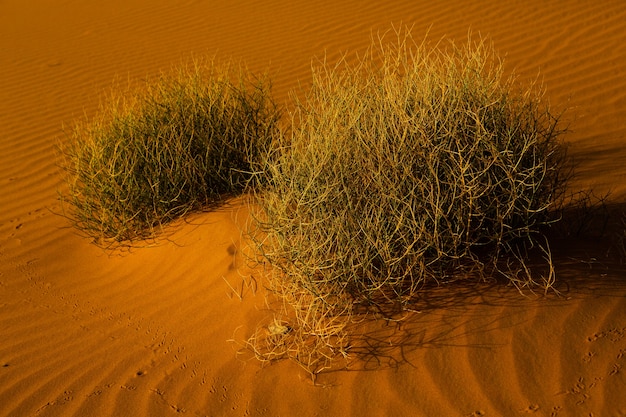The photograph captures a stark desert landscape characterized by undulating, reddish-brown sand that stretches infinitely, giving the scene an almost Middle Eastern aura. In the center, two distinct bushes, resembling tumbleweeds, serve as the focal point. The smaller bush is positioned on the middle left, while the larger, wirier bush sits to the middle right, casting a pronounced, heavy shadow to the right. The bushes display a mix of green and yellow hues, contrasting against the sandy backdrop. The sand itself is rippled with waves, adding texture to the otherwise minimalistic and barren scene. The overall color palette includes tans, shades of reddish-brown, and touches of green and yellow from the bushes, creating a harmonious yet austere visual.